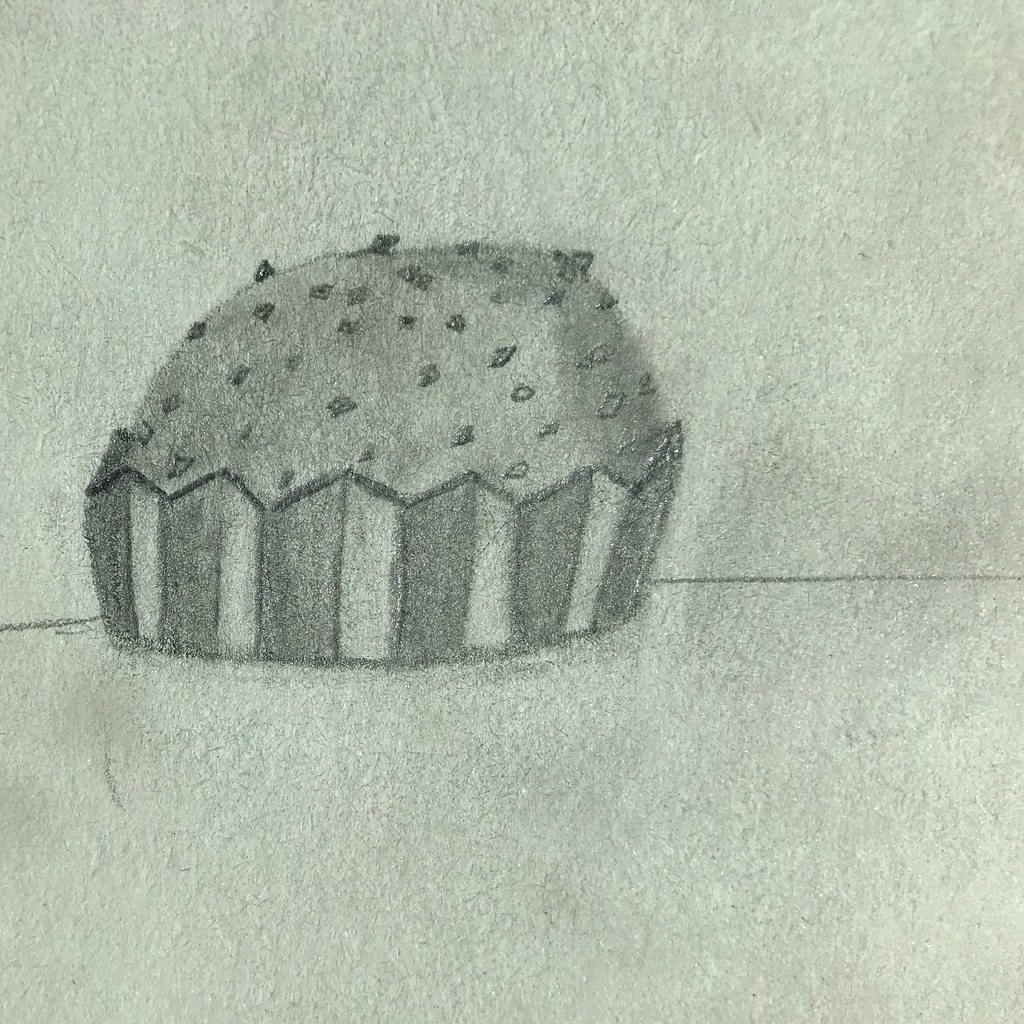This close-up photograph captures a meticulously detailed pencil drawing on a textured sheet of paper. The background is uniformly shaded with pencil strokes, revealing subtle fibers interwoven into the paper's surface. Just below the midpoint of the image, a distinct horizontal line runs across the page. Seated slightly left of center along this line is a carefully rendered depiction of a cupcake or muffin, nestled within a decorative wrapper.

The wrapper itself is adorned with vertical stripes that alternate between dark and light shades, creating a rhythmic pattern of dark, light, dark, light, continuing consistently. The upper edge of the wrapper features pointed, decorative edges, adding an ornamental touch to the otherwise simple design. The baked good perched in the wrapper rises in a dome shape, its height surpassing that of the wrapper beneath it. This dome is finely shaded to convey depth and volume, dotted with small, irregular marks that suggest the presence of chocolate chips or similar additions. Despite its simplicity, the drawing exudes careful attention to detail, capturing the essence of its subject with minimalist precision.